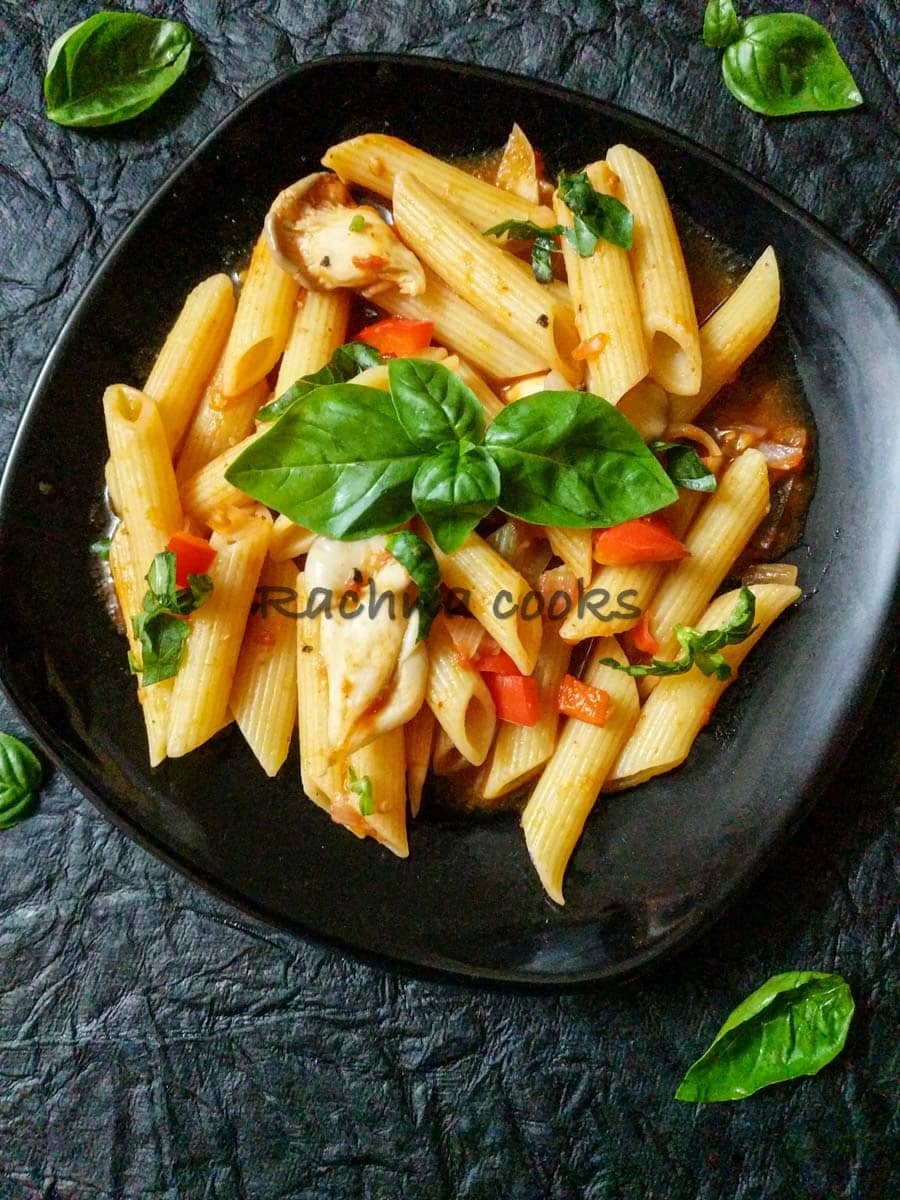Set against a textured dark gray table, this top-down portrait photograph features a black, rounded square dish centered on the table. The dish holds baked penne pasta lightly coated in a reddish-brown sauce, with thinly sliced red peppers nestled among the noodles. A sprinkle of fresh green herbs and possibly chives adds a touch of color. Four basil leaves are artfully arranged around the plate: two at the top corners, one at the bottom right corner, and another near the middle left side of the dish. A large basil leaf crowns the pasta at the center. Overlaying the image, black text reads "Rachna Cooks" superimposed at the top.